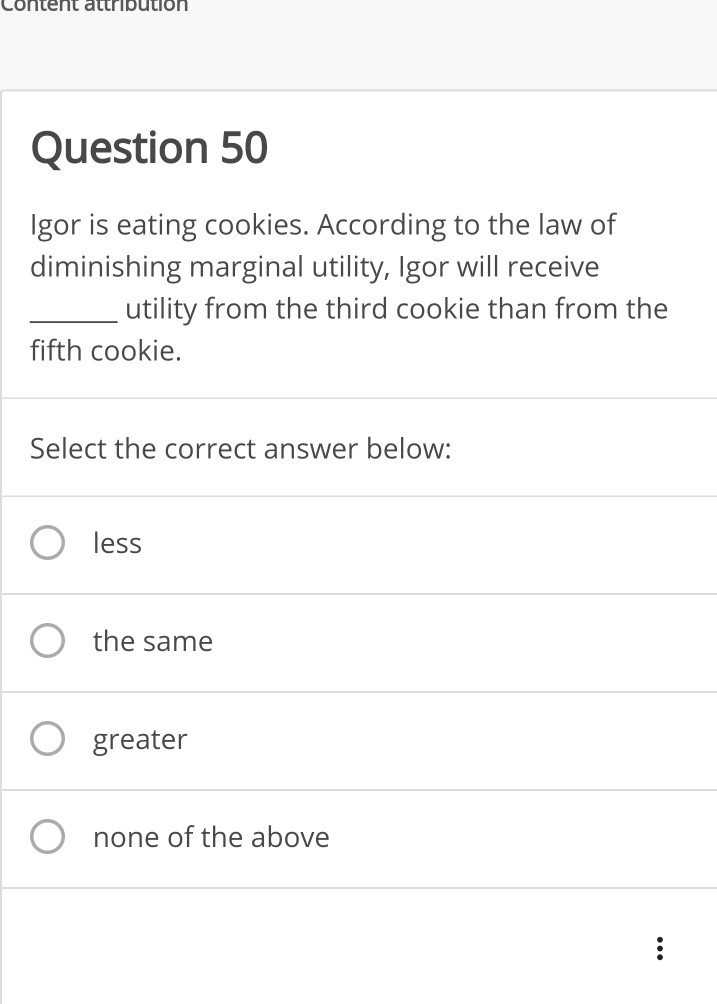Screenshot of a quiz question from a website interface. The top portion of the image shows a partially visible gray banner, cropped at the upper edges, making it unclear except for a hint that it might contain content attribution. Underneath the banner, there is a white box prominently displaying "Question 50" in bold, large font.

The question text, in a slightly smaller font, reads: "Iger is eating cookies. According to the Law of Diminishing Marginal Utility, Iger will receive _____ utility from the third cookie and from the fifth cookie."

Below the question, there are five horizontal rows. The first row, enclosed by a thin gray line, prompts "Select the correct answer below:" Following this, each of the next four rows contains a radio button on the left, allowing the user to select an answer. The answer choices are: 
1. Less
2. The same
3. Greater
4. None of the above

At the bottom right corner of the image, there is an icon featuring three vertically stacked dots, likely indicating additional options or a menu.